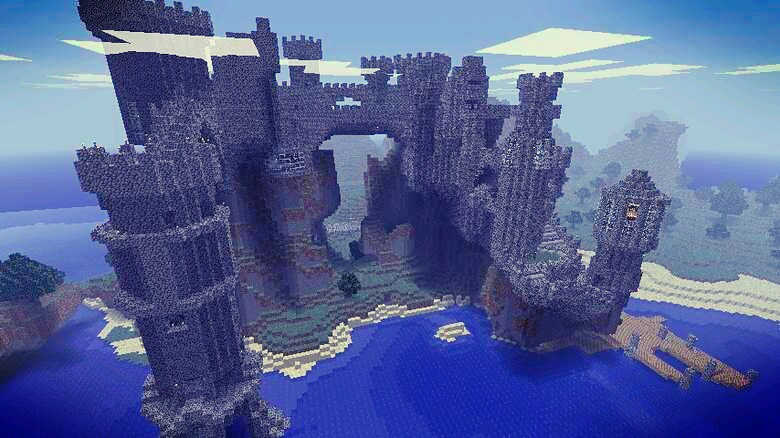The image showcases an on-screen game environment featuring a colossal gray castle majestically positioned in the center of an expansive body of deep blue water. The sky above is a serene blend of blue and light blue hues, scattered with fluffy white clouds. In the distant background, a diverse landscape unfolds with patches of verdant land dotted with trees, accompanied by additional stretches of shimmering water. A few small houses can be faintly seen amidst the greenery, adding depth to the scene. The focal point, the imposing castle, is architecturally complex, consisting of multiple layers and sections that exude an aura of grandeur and mystery.